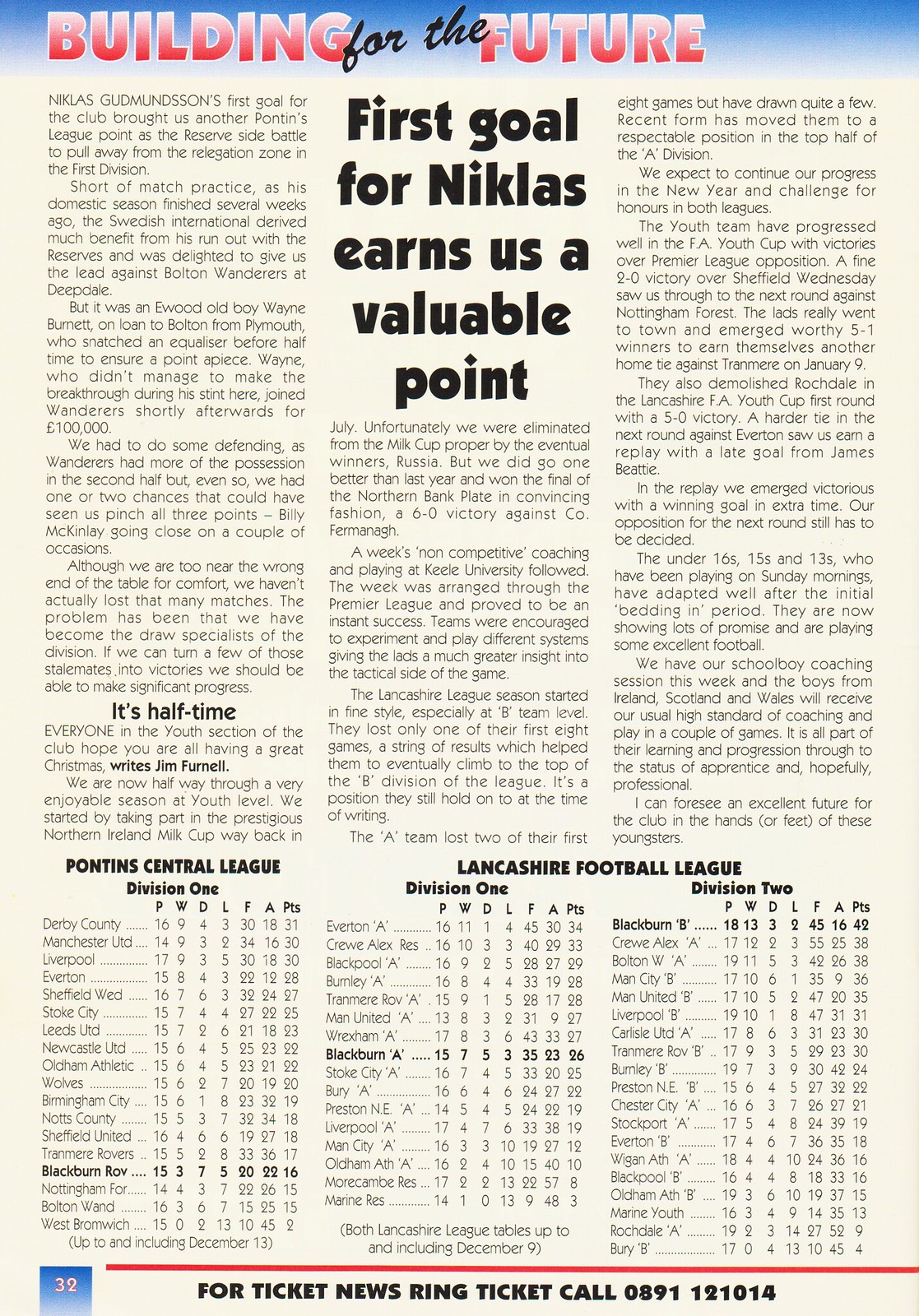The image depicts a page from a magazine or a pamphlet, characterized by a blend of colors, including light blue, blue, red, black, and off-white. At the top of the page, there is a prominent strip with a blue background, featuring the title "Building for the Future" in red and black text. Below this, centrally positioned, is a bold headline: "First goal for Nicholas earns us a valuable point." 

The primary content of the page is an article discussing football league standings, specifically focusing on the Pontus Central League Division 1 and the Lancashire Football League Division 1 and Division 2. These leagues and their respective teams are listed along with associated points. Towards the bottom of the page, there is a section that reads, "For ticket news ring ticket call 0891 121014." Additionally, a red line can be seen at the bottom of the page. The overall layout of the text extends from top to bottom and left to right, resembling a newspaper clipping or a magazine article designed with digital or press techniques.